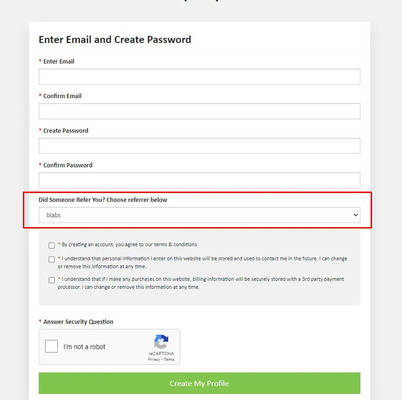The image depicts a user registration screen for creating an account. It features fields prompting the user to enter their email address and confirm it. Additionally, there are fields for entering a new password and confirming it. A dropdown menu labeled "Did someone refer you?" is highlighted with a red rectangle, emphasizing this option which allows the user to select a referrer from the menu. Below these fields, there are several checkboxes that the user must click to agree to the terms and conditions and various "I understand" statements. To complete the registration, users must also interact with a reCAPTCHA dialog box to verify that they are not a robot. At the bottom of the screen, a large, green button with white text allows users to finalize the creation of their profile.